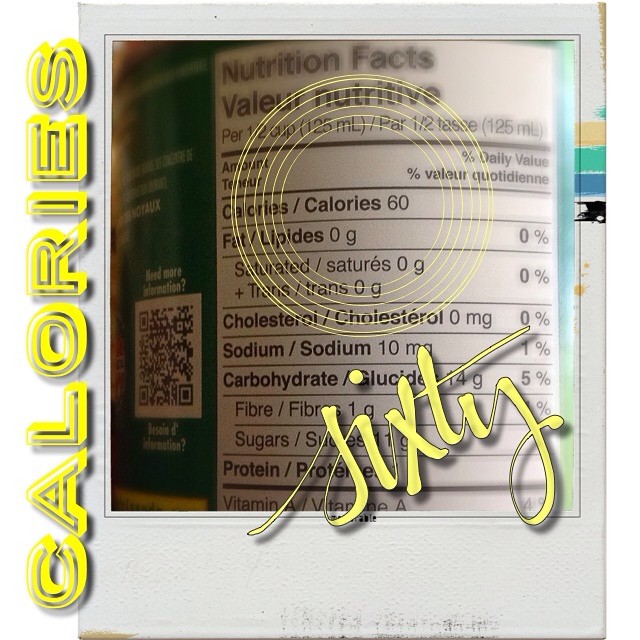This image features a vertical Polaroid photograph with the customary white border. Overlaid on the left side of the image is the word "calories," rendered in a vibrant yellow font with a distinct drop shadow, oriented counterclockwise. The focal point of the Polaroid is a close-up shot of a product's nutritional facts label, presumably from a green can of soup. The label shows standard white nutritional information, juxtaposed with a green section on the left that includes a white box designated for a barcode. Superimposed over the nutritional facts are several yellow circles, drawing attention to specific details. Below one such circle, the number "60" is prominently displayed in the same yellow, drop-shadowed, counterclockwise-oriented font. The added text and graphics appear to have been edited in using a program like Photoshop, lending a composed and stylized appearance to the image.